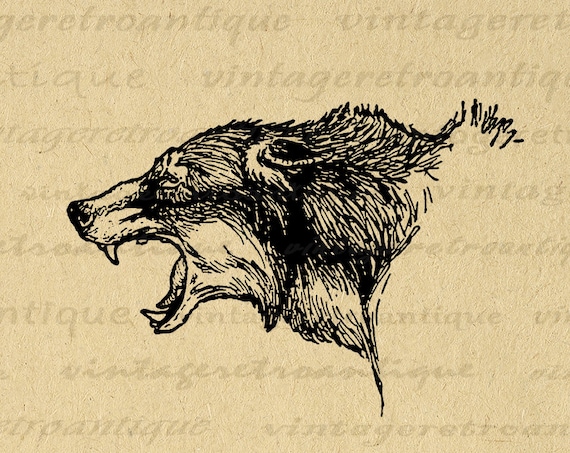This detailed ink drawing features the head of a snarling wolf in profile, facing left. The wolf's mouth is wide open, displaying its sharp upper and lower fangs, and its tongue slightly protrudes from the bottom of its mouth. It has a dark nose, a white snout and cheeks, and dark fur. The wolf's ears are laid flat against the back of its head, contributing to its fierce expression. Only the head and the beginning of the neck and back are visible; the rest of the body is not depicted. The drawing is rendered on a piece of yellowed paper, where the grain is visible. A watermark spans the background, containing the words "vintage," "retro," and "antique," written as one lowercase word in various fonts, repeated across eight rows.